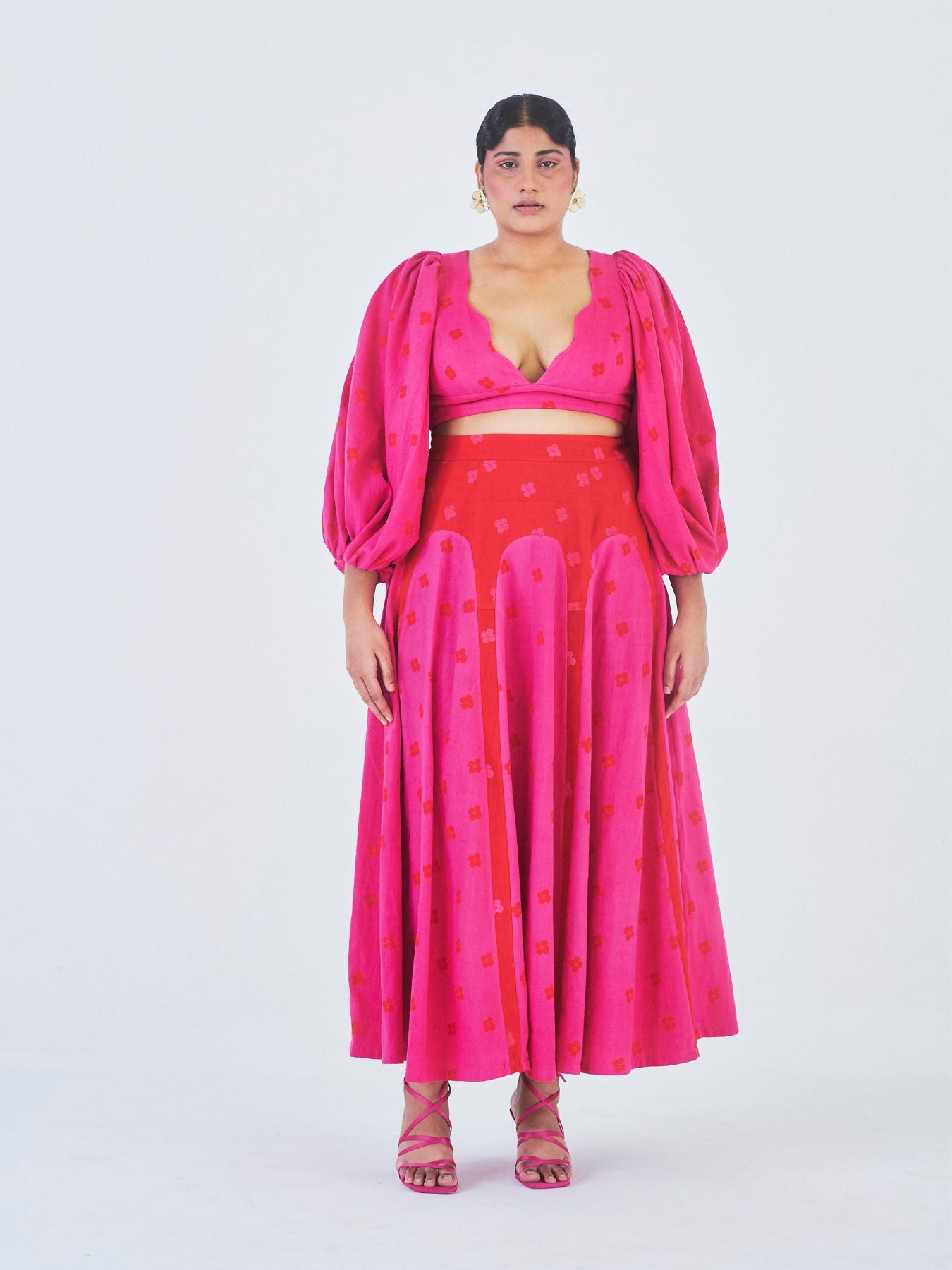The image features a woman of Indian or Middle Eastern descent, elegantly dressed in a colorful, ethnic-inspired outfit. Her attire consists of a pink top resembling a sports bra with long, flowy sleeves adorned with red diamond patterns, revealing a hint of her midriff. The ensemble continues with a mix of red and pink hues, forming an intricate design around her waist and extending into the skirt of the dress. She also wears high heels with pink straps. The woman stands centrally within the frame, her arms naturally placed at her sides, and her head positioned at the upper middle part of the image. She has dark black hair neatly parted down the middle and styled back. Her look is accessorized with two gold earrings on each ear, which dangle gracefully. The background is devoid of any text or additional objects, emphasizing the woman's striking appearance and traditional attire.